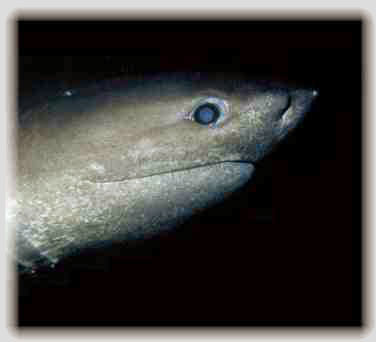The image features a framed picture with a border that is a blend of whitish and tan hues, approximately an inch thick. Within the square frame, there's a black background that accentuates the main subject: a close-up view of a shark's head emerging from the right side of the picture. The shark's head, which is grayish-tan with darker gray and black spots, occupies much of the frame, creating a sense of looming presence. The upper portion of its head appears flat with a slightly pointed, stubby nose. A distinctive white line circles around its large, circular black eye, which has a blue center. The lower jaw and mouth area of the shark is a lighter gray, with the mouth forming a long, curved line that gives the appearance of a closed mouth or a subtle, unsettling smile. The overall environment is dark, suggesting a deep-sea setting with the shark being the sole illuminated subject, emphasizing its eerie and somewhat mysterious characteristics.